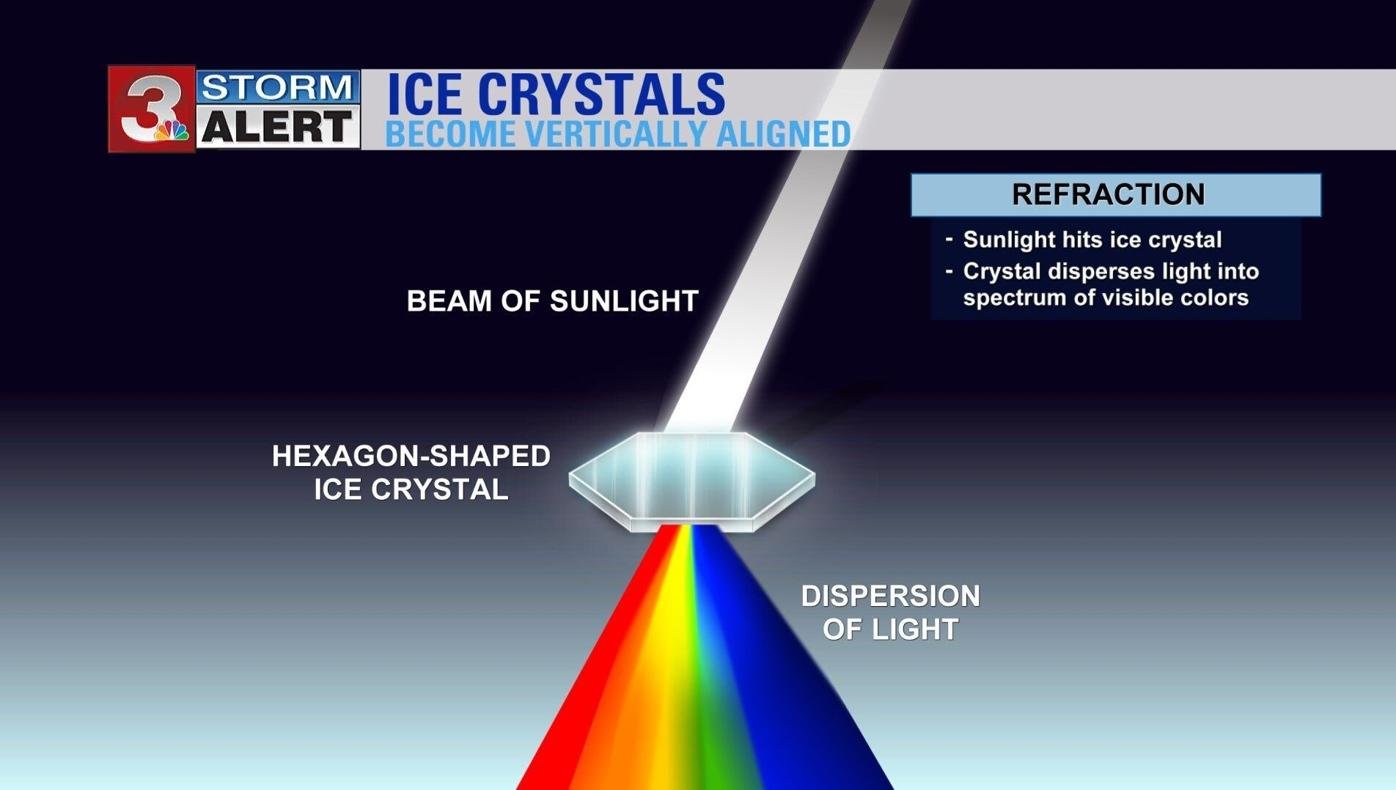This image, originally a photograph taken from a Channel 3 Storm Alert broadcast, details the phenomenon of light refraction and dispersion in vertically aligned ice crystals. The top of the image prominently features "Channel 3" in red and white, accompanied by a CBS peacock symbol, beneath the headline "Storm Alert: Ice Crystals Become Vertically Aligned." The central focus is a scientific diagram illustrating the process: a beam of sunlight, depicted in white, strikes a hexagon-shaped ice crystal. Notably, rainbow-colored beams—in red, yellow, green, and blue—are shown entering the ice crystal. As light exits, it disperses into a spectrum of visible colors. On the right side, captions in all capital letters read "Dispersion of Light" and delve further into the details of light behavior, stating "Refraction: Sunlight Hits Ice Crystal. Crystal Disperses Light Into a Spectrum of Visible Colors." This visual elegantly explains how light interacting with ice crystals can result in a natural display of rainbow colors in the sky.